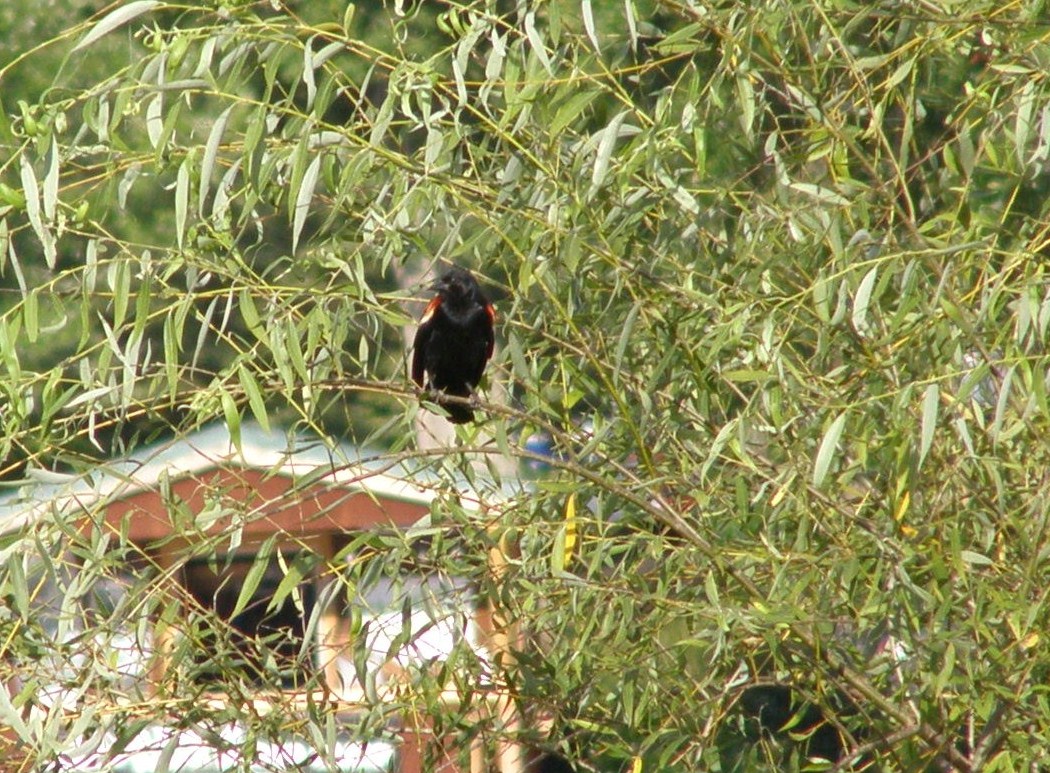The photograph captures an outdoor setting almost entirely covered by the branches of a small tree with long, thin green leaves. Perched on one of these branches is a black bird with distinctive red, white, orange, and yellow tips on its wings, looking to the left. The bird, which has a very short beak, is the focal point of the image. In the blurred background, a white building with a partially red roof and wooden trim is visible, featuring a window underneath the roof. The scene is brightly illuminated, indicating it is daylight, though no sky is visible.